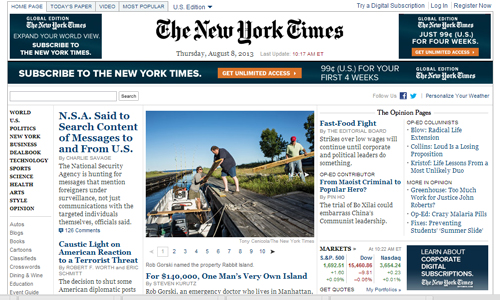The image depicts a zoomed-out view of The New York Times website as it appeared on Thursday, August 8, 2013. Prominently displayed at the center top is the text "The New York Times" in black lettering. Flanking the title, on the left side, is a black square with some writing, mirrored on the right by another black square with an orange rectangle at the bottom, resembling a clickable button.

Above the main title, on the left, are five categories written in blue, while three categories including a 'login' option, appear on the right. Directly below "The New York Times" header, a subscription prompt reads, "Subscribe to the New York Times," accompanied by an orange rectangle labeled "Get unlimited access." To its right, a promotional offer states, "99 cents for your first four weeks."

Beneath the subscription prompt is an article titled, "NSA Said to Search Content of Messages to and from US." Centrally located on the page is an image depicting a scene of two individuals on a dock; one appears to be working on something while the other holds lumber. The background features a clear blue sky and trees, indicating an outdoor setting.

Search results seem to be displayed in a sequence from one to ten. Additionally, two more articles are positioned to the right of the central image, each with blue hyperlinks. The entire page maintains a clean, white background.